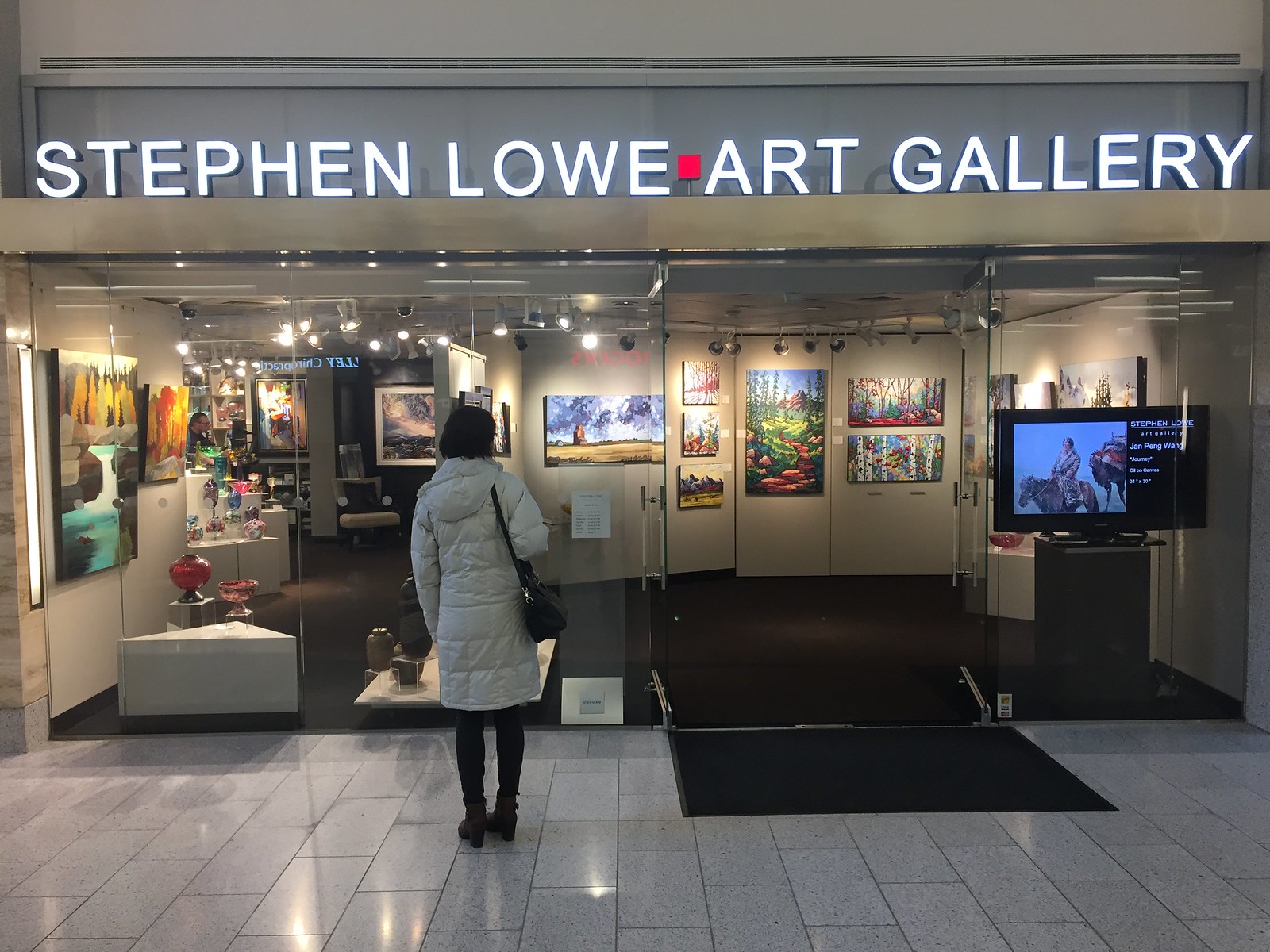The image showcases the front of the Stephen Lowe Art Gallery, situated inside what appears to be a shopping mall. The gallery entrance is framed by large glass walls and double glass doors, which are open, inviting viewers to look inside. Above the entrance, a prominently lit white sign displays the name "Stephen Lowe Art Gallery." 

Standing outside the gallery is a woman dressed in a white puffy long coat, paired with skinny black jeans and boots. She carries a black leather bag over her right shoulder. She stands on a tile floor, complemented by a large black rug placed near the entrance. 

Inside the gallery, the walls are adorned with numerous paintings and portraits. To the left, some pieces of pottery and glass artwork are arranged on white platforms beneath the paintings. A TV screen to the right of the entrance showcases detailed information about an exhibit, specifically highlighting an oil canvas painting titled "Journey" by Jan Peng Wang. This painting depicts a Native American on a horse. The carefully curated art pieces and the inviting ambiance from the glass facade create a welcoming atmosphere that draws attention even from outside.